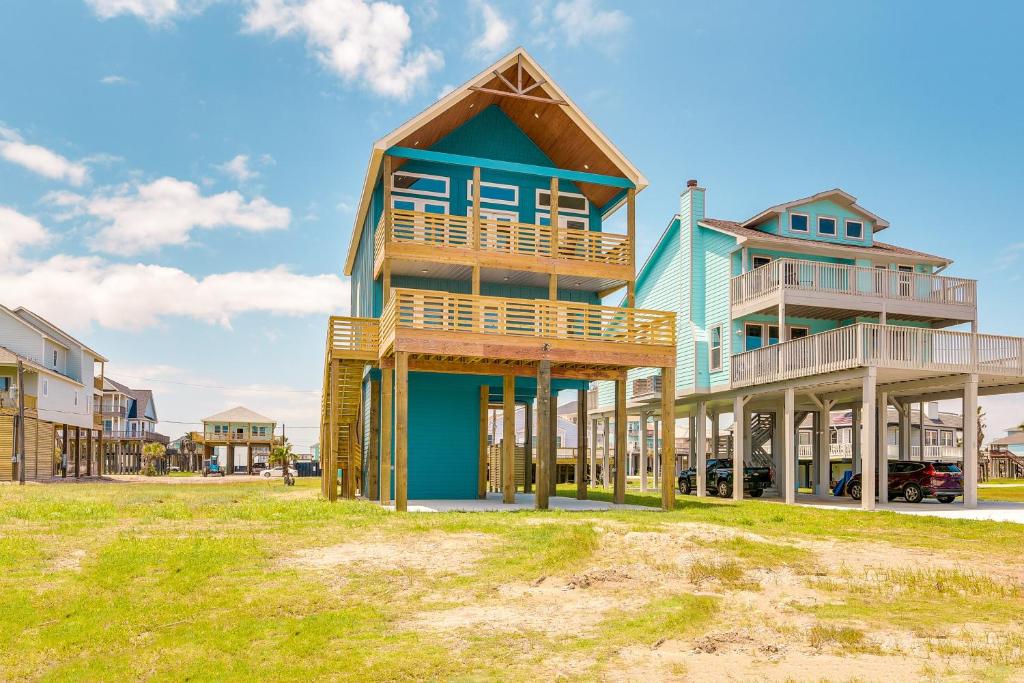In this vibrant outdoor scene, the bright blue sky, adorned with a few thin clouds floating on the left, sets a picturesque backdrop. Prominently displayed are beach homes raised on wooden stilts, likely a precaution against potential flooding or a nearby ocean. Centered and to the right, the turquoise-colored home features a light grassy front yard mingling with whitish sand, accentuating its beachside setting. It flaunts a new, tan wooden deck, adding a touch of modernity. Adjacent, the white house showcases a matching white deck and railing. Below the homes, cars are conveniently parked, with a black truck and SUV visible beneath the white house. The distant background reveals more stilted homes, with the farthest being white and another nearby in an off-blue hue, both keeping with the coastal architecture. The scene is bathed in sunlight, highlighting the lively and serene atmosphere of this beachside neighborhood.